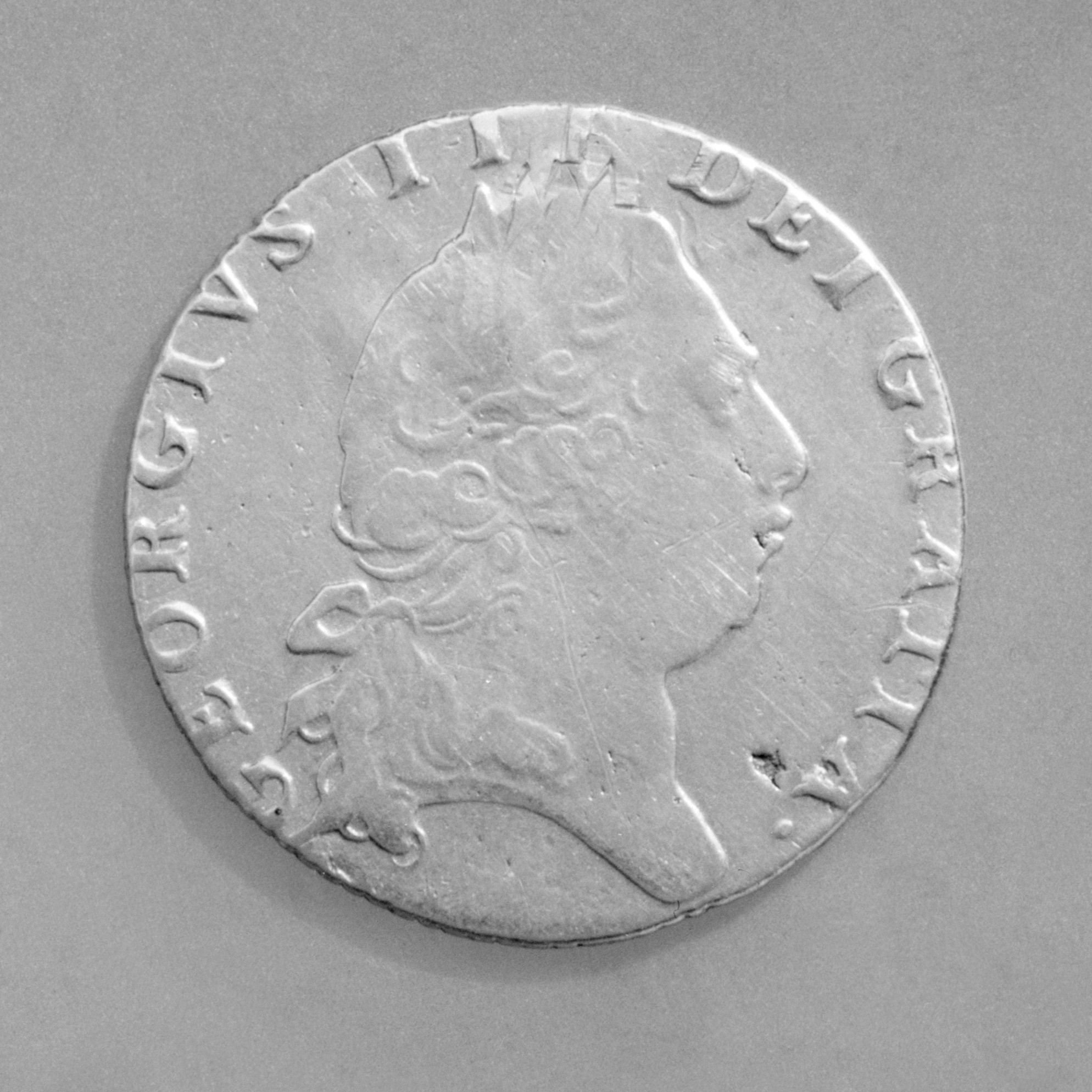This image features an old, matte silver coin with the portrait of a historical figure on its front side, set against a solid gray background. The coin appears to be round and noticeably lacks a rim, making it resemble a flat piece of silver. The central image is a side profile of a person adorned with a wig styled in curls, reminiscent of colonial times, looking to the right. The figure, whose gender is ambiguous, appears to be significant, possibly a dignitary. The text around the coin’s circumference, written in Roman numerals, reads "George IV" and is accompanied by additional letters that appear to spell out "D-E-L-L-E-G-H-A," suggesting it might be of Italian origin. The coin's dull, unpolished surface gives it a unique, almost clay-like appearance, which blends subtly with the background.